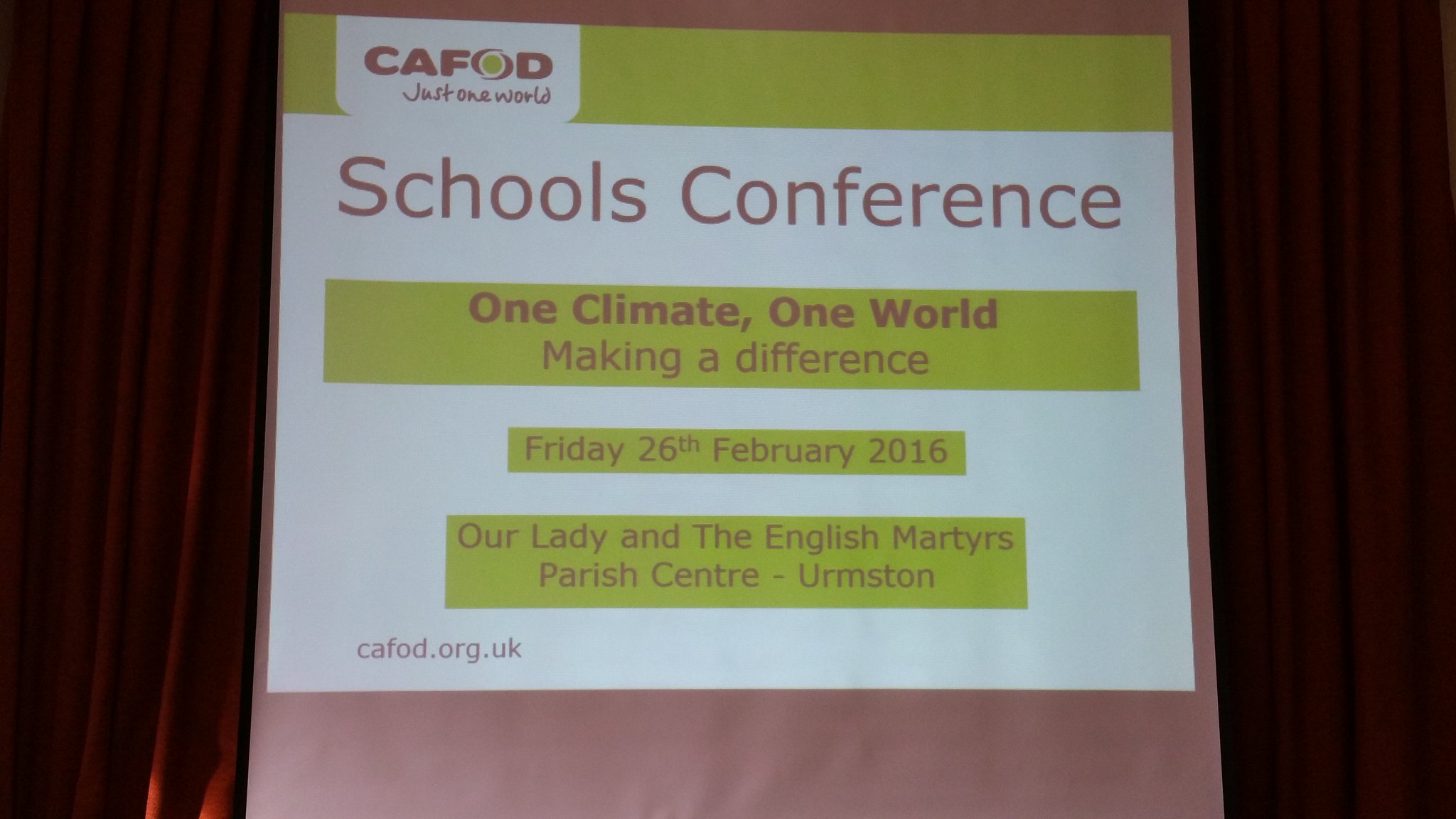The image shows a detailed color sign projected on a wall with text in black on a white background, accented by areas of green. The sign features a logo at the top that reads "CAFOD," with "Just One World" beneath it. The main text states "School Conference: One Climate, One World, Making a Difference," and provides details for the event: "Friday, 26th February 2016," at "Our Lady and the English Martyrs Parish Centre, Urmston, cafod.org.uk." The edges of the projection are framed by large stage curtains, adding to the formal setting. The overall scene suggests a focus on climate change, church activity, and educational initiatives.